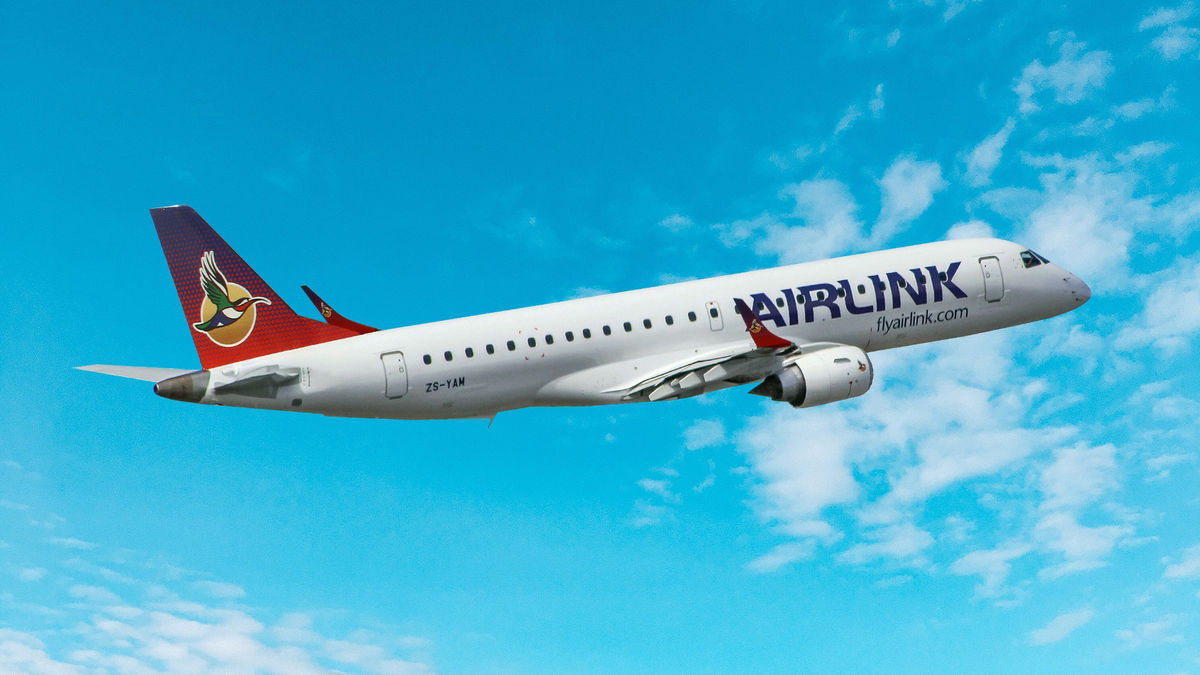This image features a prominently white airplane flying mid-flight against a backdrop of a blue sky with scattered white clouds. The airplane showcases the word "Airlink" in dark blue letters, with "Flyairlink.com" written just below it on the right side. Toward the rear, the registration "ZS-YAH" is visible. The tail of the plane displays a vibrant gradient design that starts as red at the bottom and fades to purple at the top, featuring a colorful bird logo. The bird has green wings, an orange chin and beak, and its body is white with shades of gray or blue. The plane appears to be flying from left to right, centered in the image.